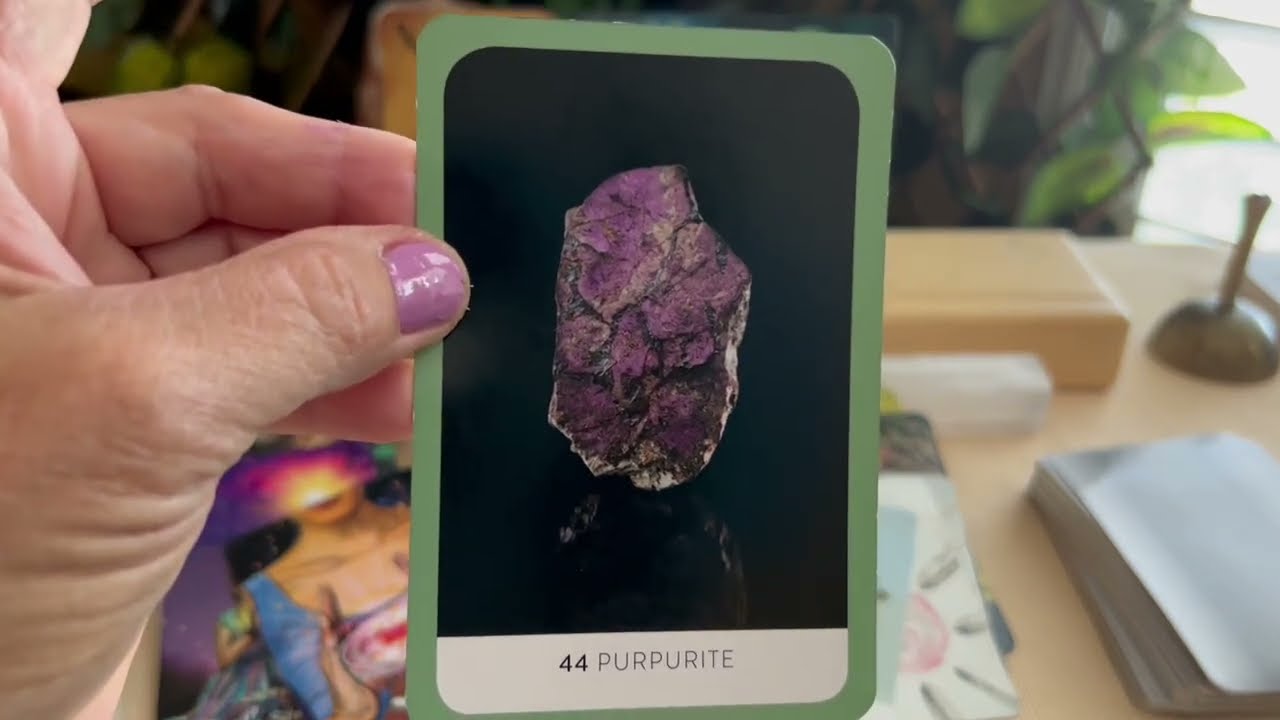The image is a detailed photograph of a woman's hand with light pink nail polish, prominently holding a vertically oriented card in the center. The card, bordered in green with a black background, displays an image of a purplish gem or rock at its center. Below the image, in a white bar, is the text "44 Purpurite," suggesting the card is part of a game or collection. The hand is positioned towards the left of the frame, using the thumb, middle, fourth, and pinky fingers to hold the card. The background is blurred, revealing a beige wooden desk that spans the width of the photo, accompanied by indistinct objects such as curtains, drapes, or possibly plants. The setting appears to be an indoor house or office, captured during daytime. The photograph is rich in colors, including purple, green, black, white, and various shades of beige and pink.